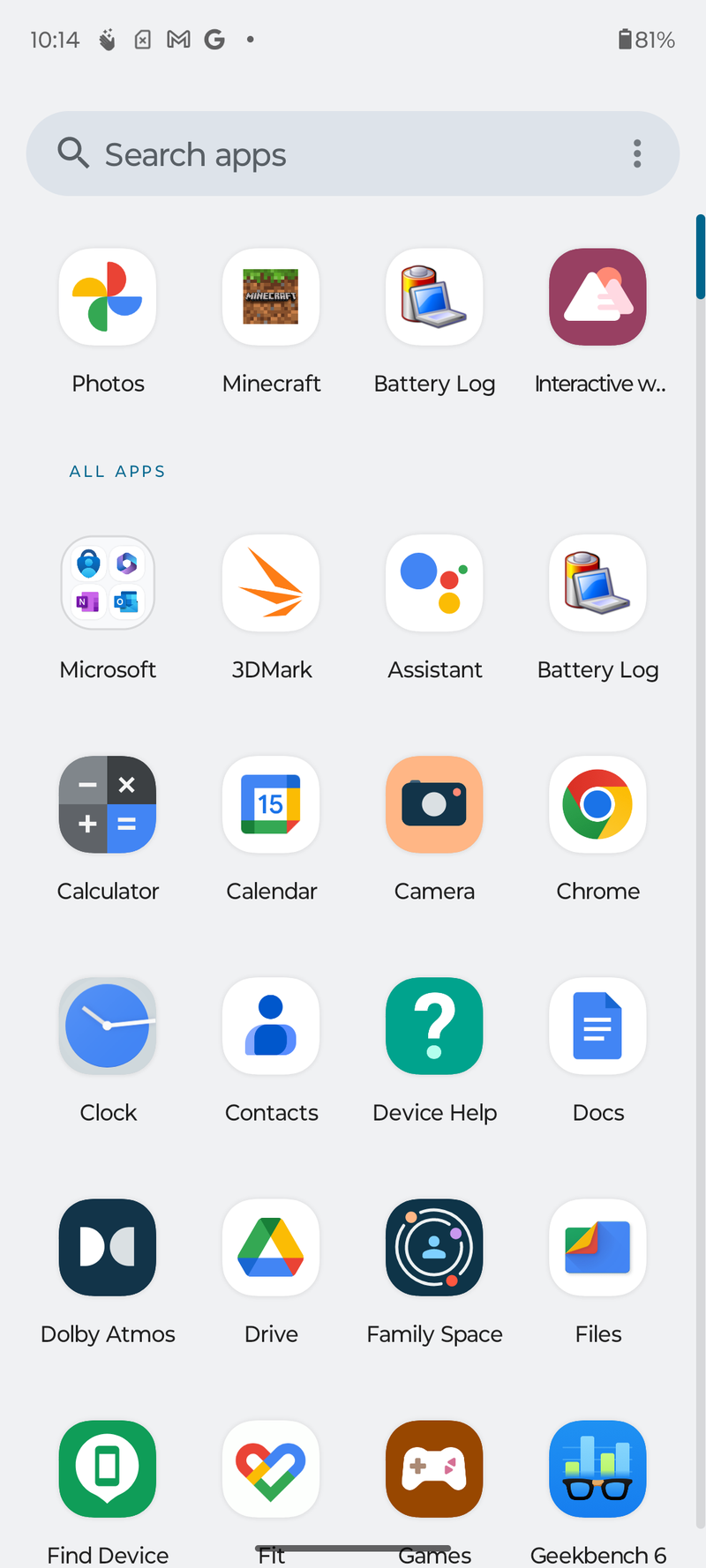This is a detailed description of a smartphone screenshot displaying its home page. At the top of the screen, the time is shown as 10:14 AM, accompanied by a series of icons. Notably visible are the Gmail and Google icons, with the battery icon on the far right indicating an 81% charge. Directly below this is a search bar labeled "Search apps." 

On the home page, there is a row of four app icons, listed from left to right: Google Photos, Minecraft, Battery Log, and Interactive Widget (the full name is obscured). Below this row, there is a light gray area where it says "All apps." Here, app icons are arranged from left to right as follows: Microsoft, 3D Mark, Assistant, Battery Log (listed again), Calculator, Calendar, Camera, Google Chrome, Clock, Contacts, Device Help, Documents, Dolby Atmos, Google Files, Find Device, Google Fit, Games, and Geekbench 6. Each app is represented by an icon consistent with its function.